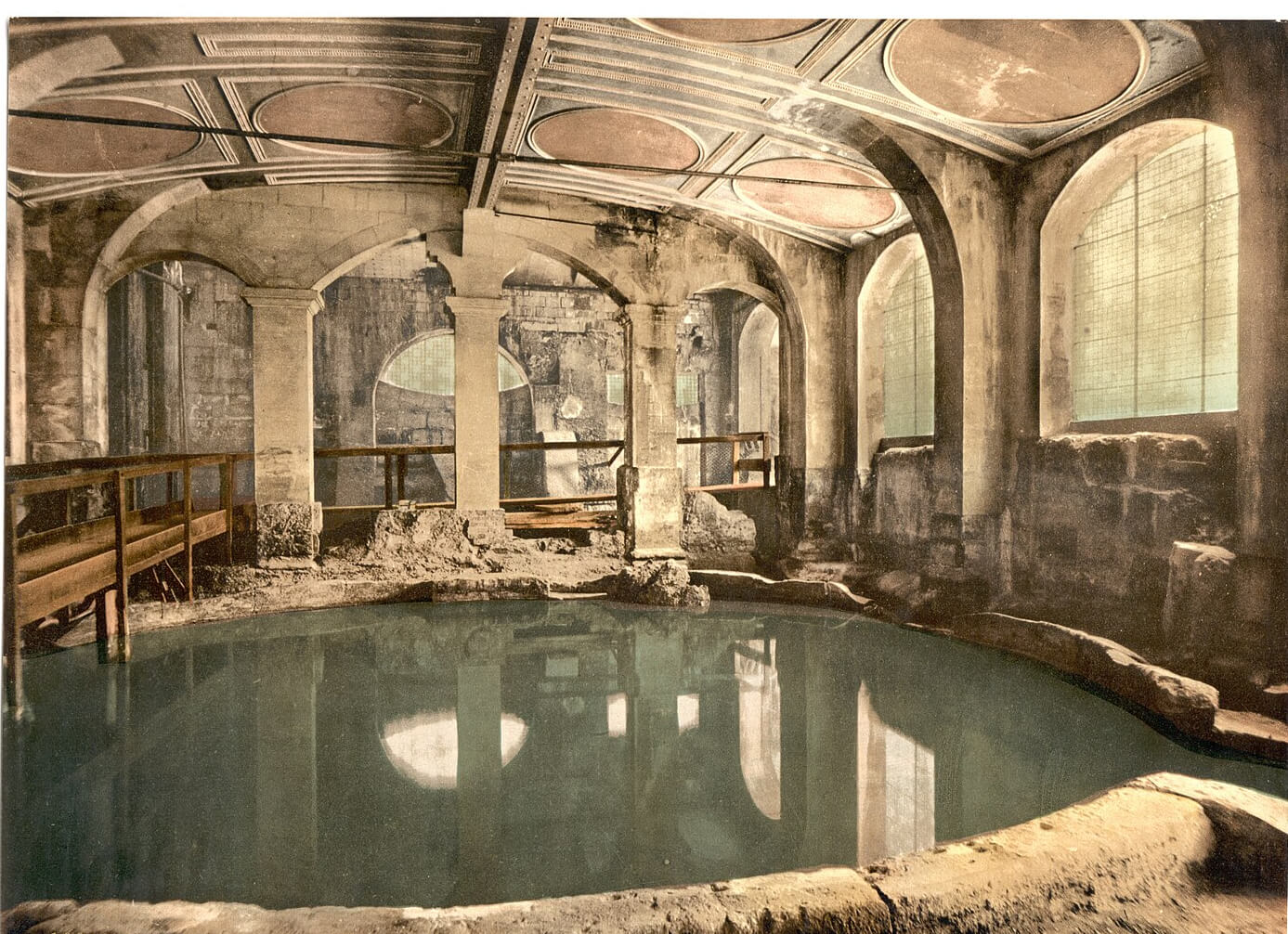The image depicts the interior of what appears to be an ancient bathhouse or indoor pool, reminiscent of a Roman bathing structure. The central feature is a circular pond or pool surrounded by a stone edge made of grayish-brown stone blocks. This stone edge runs from the bottom left of the image, enclosing the pool, and transitions into a channel that exits the image at the bottom right.

Three stone pillars, which also appear to be composed of grayish-brown stone blocks, are positioned on the top side of the pool. Above the pool, on the left side, a wooden bridge with a dark wood guardrail stretches across the waterway, extending from the left middle of the image and disappearing behind the pillars, eventually exiting through an archway doorway on the right.

The ceiling, slightly visible in the image, features an Art Deco design with large circular patterns and includes a steel I-beam complete with rivets, which attaches to one of the central stone pillars. The pond's water has a murky green hue, adding to the ancient ambiance of the setting.

Numerous large, oval-topped windows with pillars between them frame the right side, allowing light to reflect off the water, contributing to the bathhouse's serene atmosphere. The scene is completed by the presence of an intricate ceiling design with circular elements and large round circles with pink spots, enhancing the historical and architectural depth of the bathhouse.